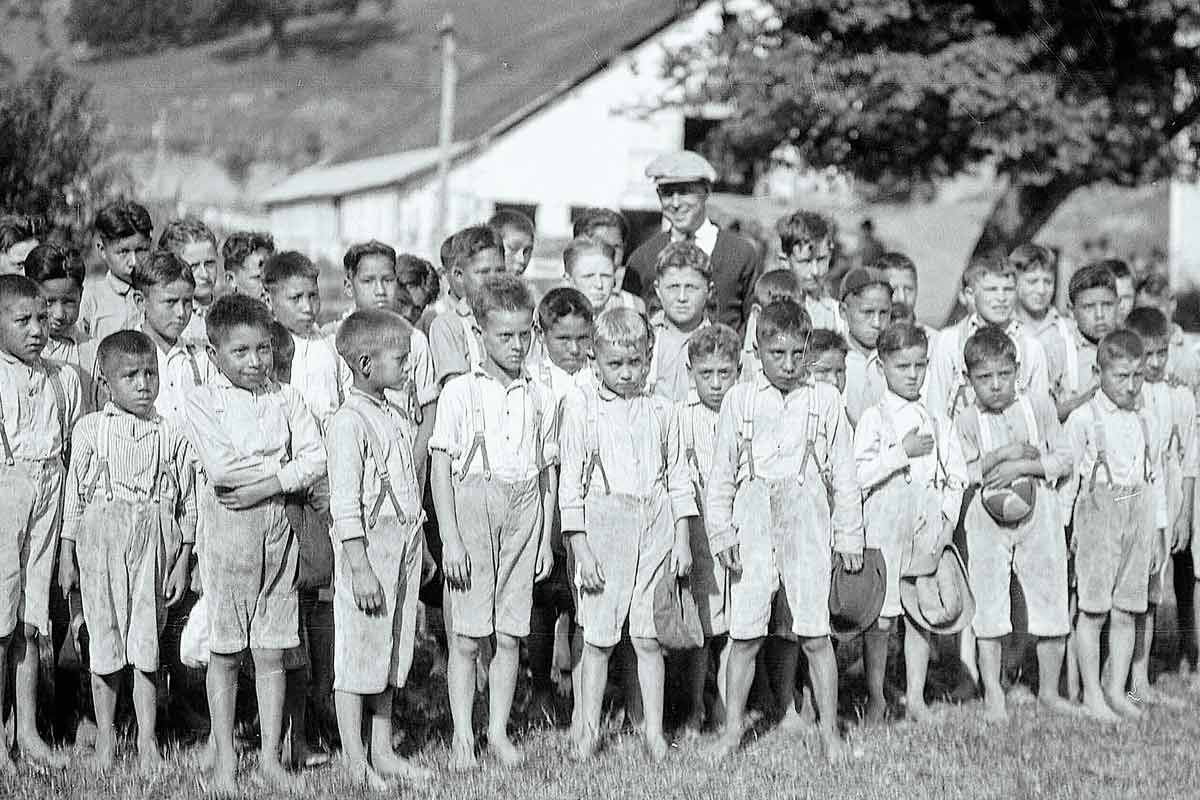This is a vintage black-and-white photograph, likely taken in the early 1900s, featuring approximately 50 young boys aged between 4 to 7 years old. The children are gathered outdoors, possibly in a schoolyard, as indicated by the rustic building and tree visible in the background. Each boy is identically dressed in knee-length shorts with suspenders and long-sleeved, white collared shirts. Most of them are barefoot, with some rolling up their sleeves to contend with what appears to be a warm, sunny day, as evidenced by the shadows cast on the ground. Many of the boys have their hands on their chests, which could suggest they are participating in a pledge or singing the National Anthem. Standing behind them is an older gentleman, perhaps in his 40s, possibly a teacher or mentor. He is dressed in a blazer or cardigan, a tie, and a vintage-style chimney sweeper hat. The boys, all sporting short haircuts, are facing attentively to the right of the photo.